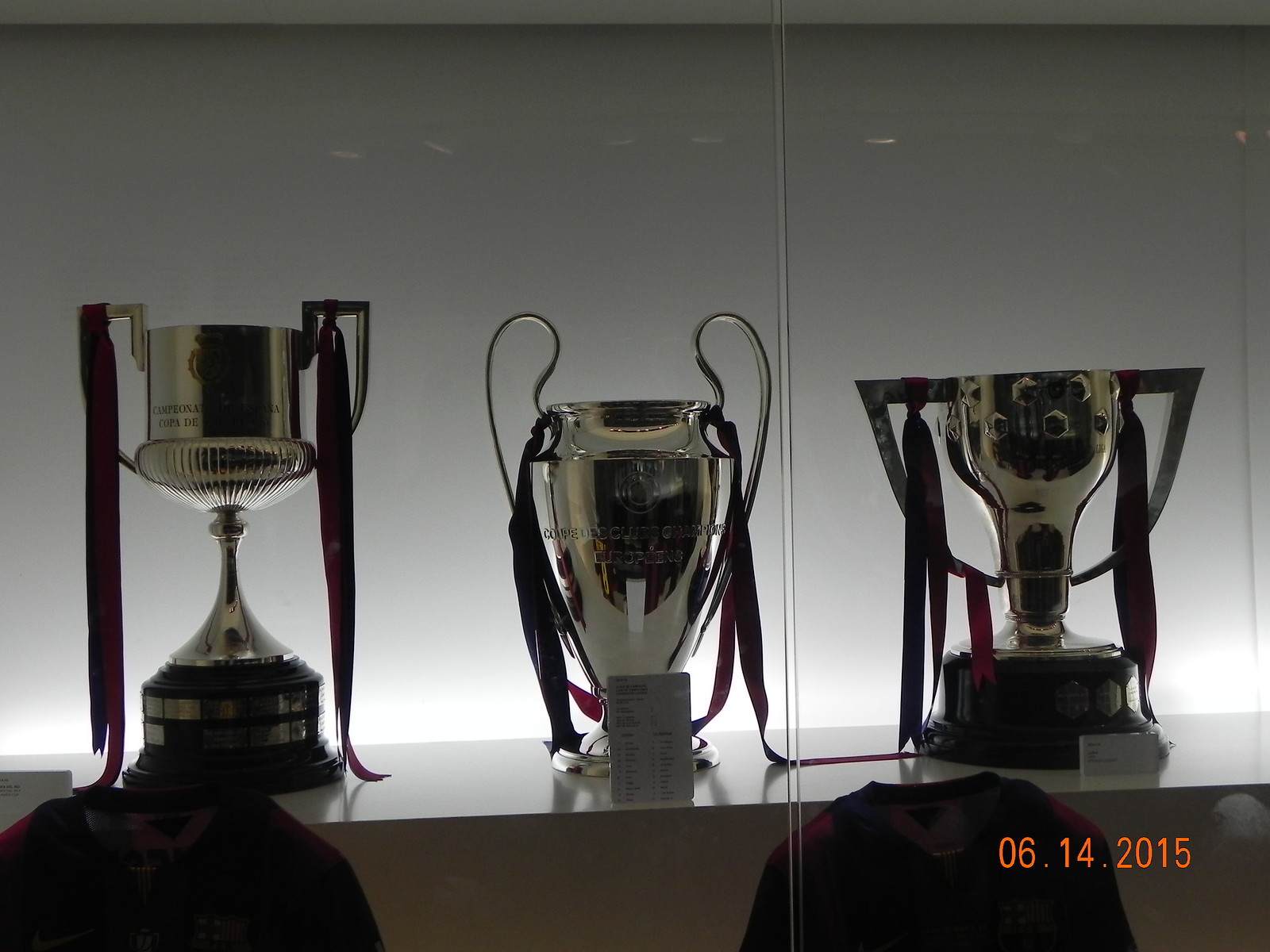This photo, taken on June 14th, 2015, depicts three distinctive trophies displayed inside a glass case with a white background and backlighting that highlights their features. The first trophy, positioned on a broad, circular black base, boasts a long neck and cup-like design with ribbons hanging from either side. The second trophy, resembling a substantial cup or vase, is adorned with large handles extending past the vessel and has something potentially written or attached in front of it. It also features ribbons on both sides and sits on a proportionate base. The third trophy resembles an oversized chalice or wine glass with an upside-down half-circle design and handles, also accompanied by ribbons. Alongside the trophies, there appear to be other items on the next shelf, possibly clothing like jerseys or sweatshirts. The image, rendered in black and white, includes an orange date stamp in the corner that reads "06-14-2015."